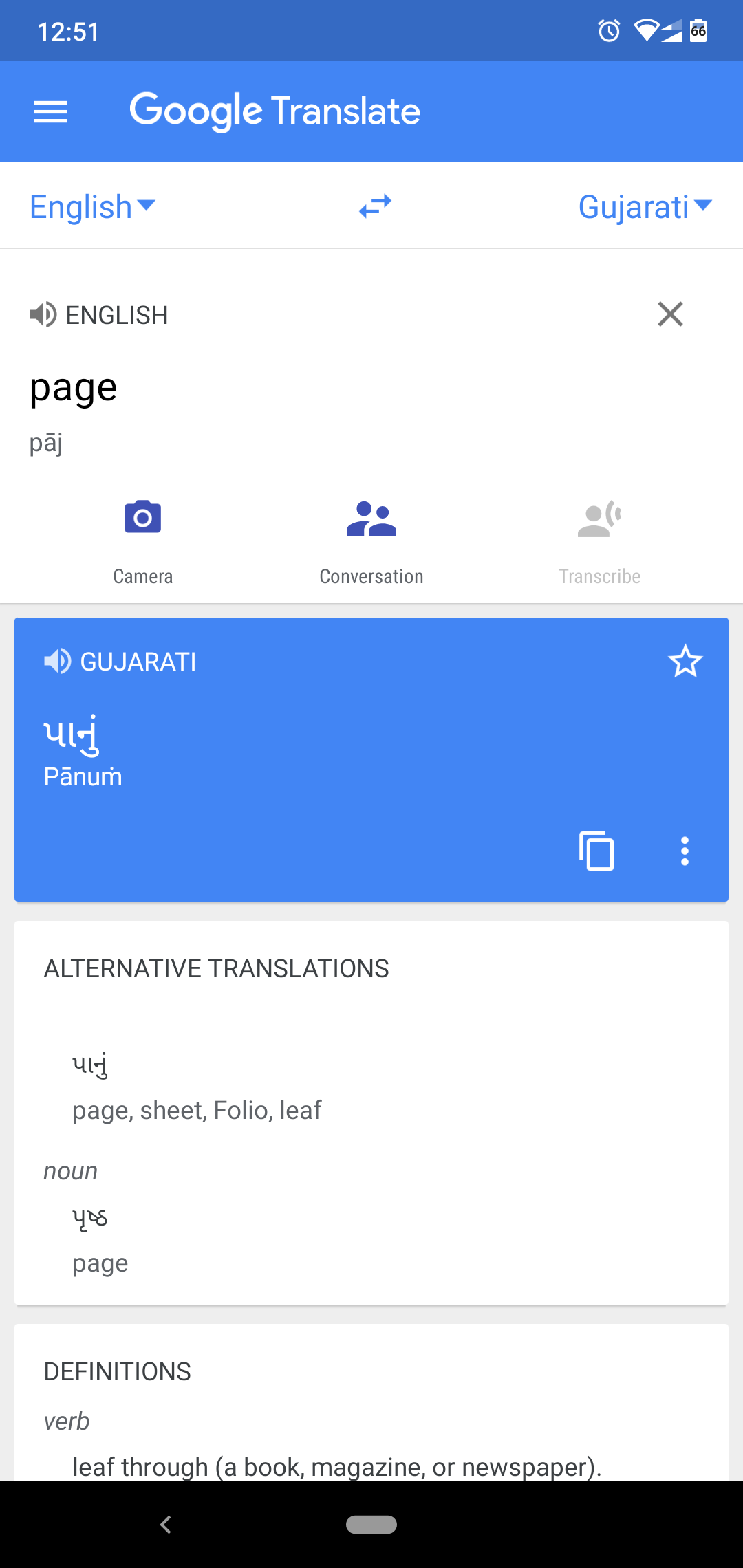Screenshot of the Google Translate app interface displaying both English and Gujarati languages. The top of the screen shows "1251" and a hamburger menu icon. The translation direction is set from English to Gujarati, indicated by a rightward arrow above and a leftward arrow below the languages. 

In the main translation space, the English word "page" is provided and its pronunciation in Gujarati (G-U, J-A-R-A-T-I) is noted. Below this, there is a blue-highlighted "camera" icon next to "conversation," "transcribe," and "conversation and camera."

Further details in the interface include the Gujarati translation accompanied by a speakerphone icon, a star icon, and what appears to be Arabic or another script. Underneath, another transliteration "P-A-N-U-M" is displayed, followed by icons of two squares and three vertical dots.

The section labeled "Alternate translations" presents multiple options for the word "page," including "sheet," "folio," "leaf" (noun), and "definitions" such as "leaf through" (in parentheses, indicating usage with a book, magazine, or newspaper).

At the very bottom of the screen, a black rectangle contains a gray arrow pointing to the left alongside a gray bar in the center.